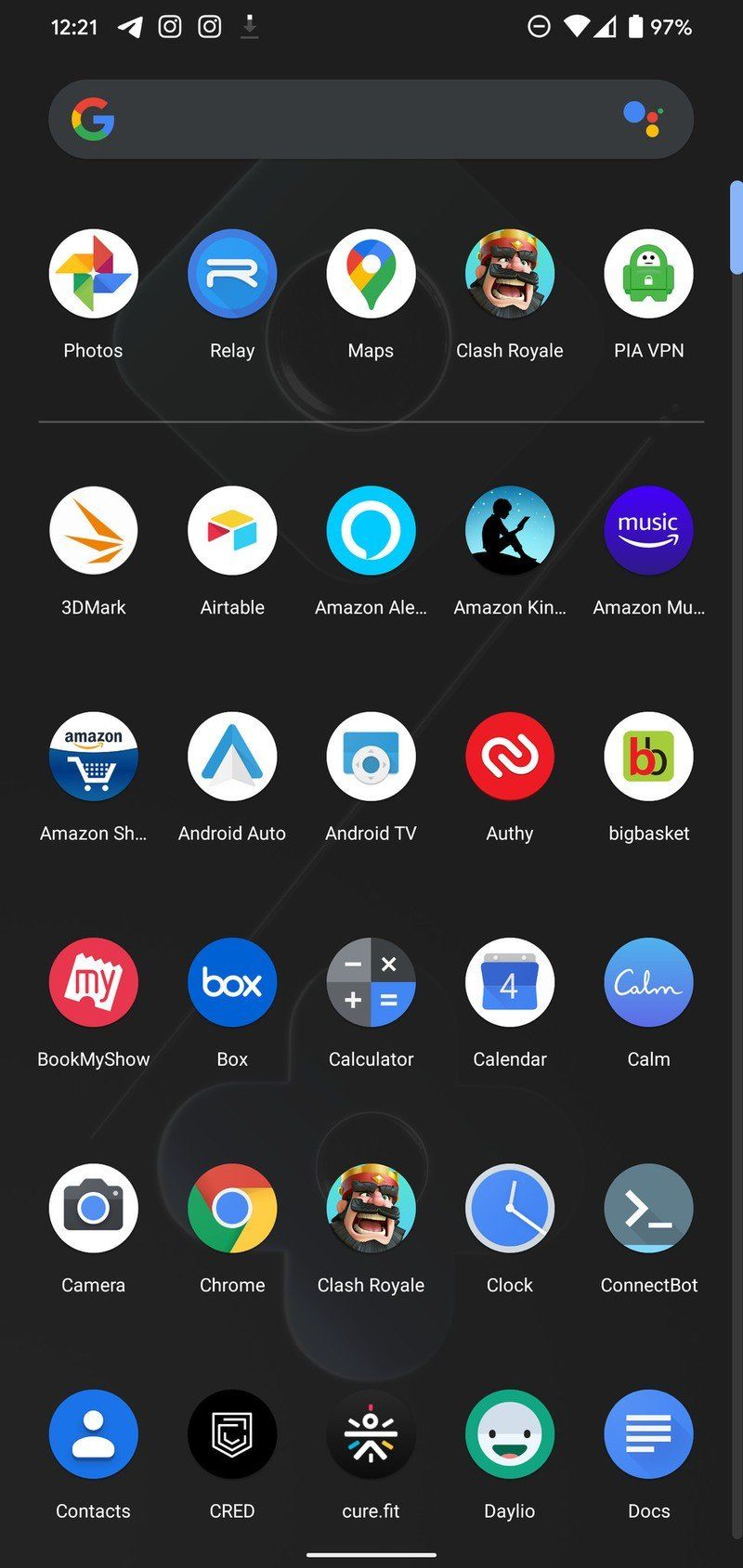A detailed snapshot of a smartphone screen set to dark mode, highlighting various system stats and a comprehensive collection of apps. The background is black, accentuating the white and colored icons. At the top of the screen, it’s 12:21 PM, with a strong signal, connected to Wi-Fi, and a battery charge of 97%. Below these indicators, a Google search bar sits prominently.

The main display shows six rows of apps, each consisting of five icons:

1. **First Row**:
   - Photos
   - Relay
   - Maps
   - Clash Royale
   - PF VPN

2. **Second Row**:
   - March 30 (possibly a calendar event or app)
   - Airtable
   - Amazon Alexa
   - Amazon Kindle
   - Amazon Music

3. **Third Row**:
   - Amazon Shopping
   - Android Auto
   - Android TV
   - Authy
   - Big Basket

4. **Fourth Row**:
   - Book My Show
   - Box
   - Calculator
   - Calendar
   - Calm

5. **Fifth Row**:
   - Camera
   - Chrome
   - Clash Royale (appears again)
   - Clock
   - Connect Bot

6. **Sixth Row**:
   - Contacts
   - CRED
   - CureFit
   - Daylio
   - Docs

This image provides a meticulous overview of the user’s organized home screen, capturing a moment in their digital life.